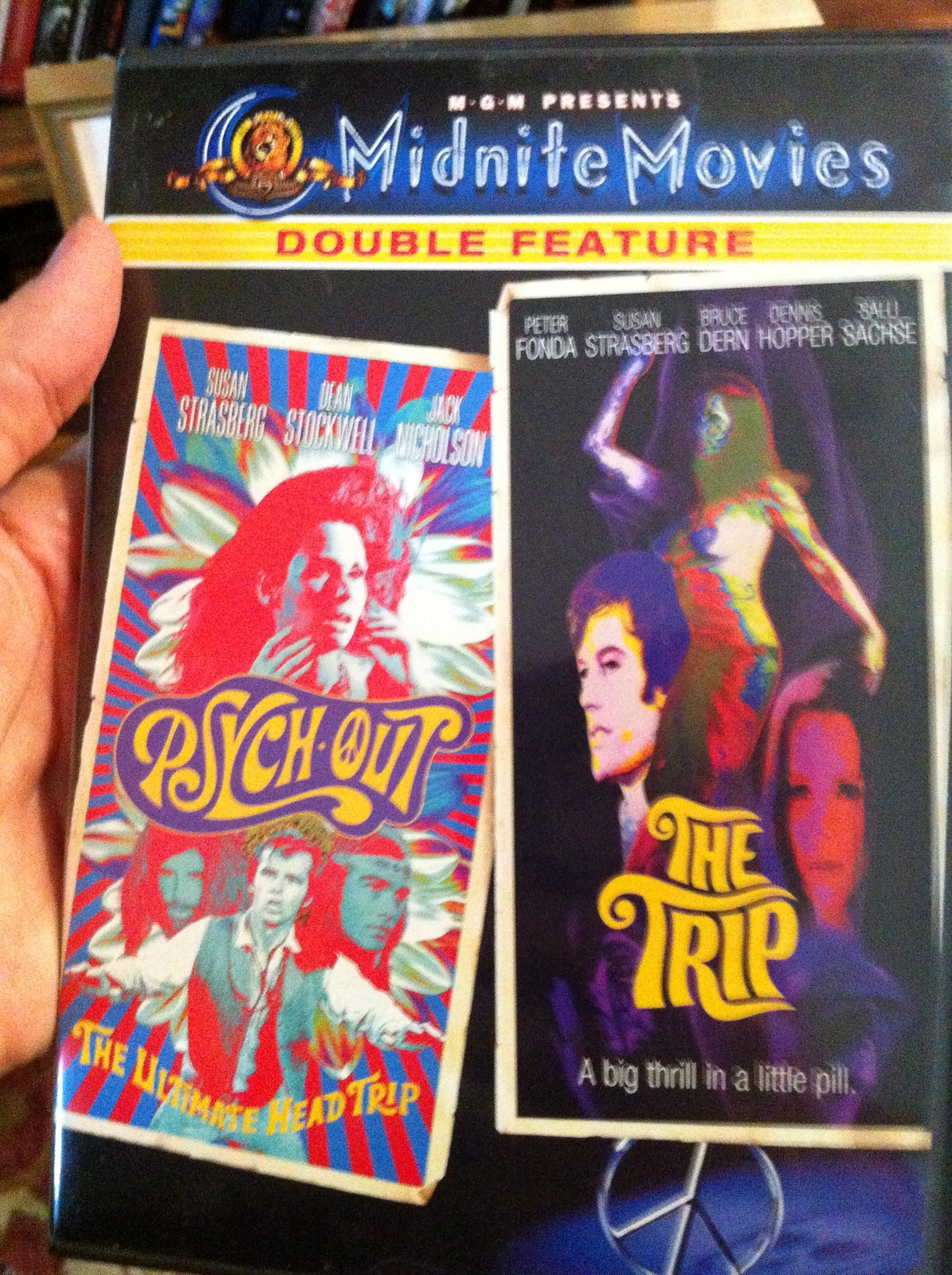A vertically aligned rectangular image showcases a person’s left hand holding a DVD cover featuring a classic "Midnight Movies" double feature from MGM. The DVD cover, set against a yellow background, prominently displays the iconic MGM lion logo with the text "MGM Presents" in blue and white. Below this, in yellow capitalized letters against a red bar, it states "Double Feature."

The left side of the DVD cover highlights the film "Psych Out," starring Susan Strasberg, Dean Stockwell, and Jack Nicholson. The movie is described as "The Ultimate Head Trip," with artwork evocative of a 1967 poster. The cover features an eclectic design with a prominent red and white flower backdrop, rays of red and blue emanating outward, and a woman with her hands raised to her face. Below, a male figure is flanked by two women, all set against a purple background.

On the right side, the cover showcases "The Trip," featuring Peter Fonda, Susan Strasberg, Bruce Dern, Dennis Hopper, and chilling eyes looking out towards the viewer. The tagline, "A Big Thrill in a Little Pill," hints at its psychedelic theme. The artwork portrays a woman in a red dress and headband, her arm raised, next to Peter Fonda, who appears in a white shirt with a red and blue vest and an open collar. Below, another woman with a blank expression completes the visual. A silver peace symbol against a blue background and modeled patterns highlights the counter-cultural essence of the films.

Both film covers are bordered in white, adding a classic touch to their vibrant and distinctive 60s-inspired designs.